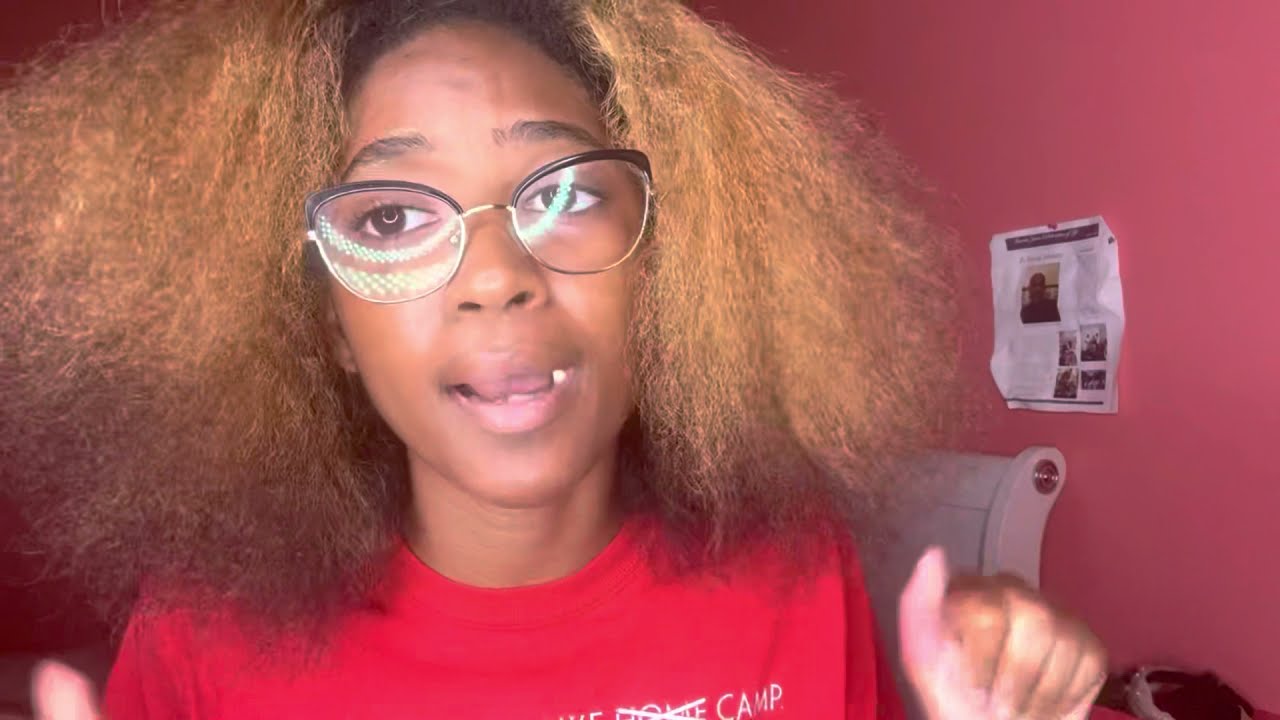In the image, a Black woman with shoulder-length, curly, caramel-orange hair appears to be engaged in a video chat or FaceTime call, as suggested by the reflection visible in her black-rimmed glasses. Her hair, slightly frizzy and seemingly dyed, frames her face, accentuating her full, dark eyebrows and deep brown eyes. The woman is wearing a red t-shirt with white lettering that reads "blah [crossed out] camp" and is sitting on an arched, white wooden chair in a room with pink walls. She has her left hand raised, with her fingers pointing outward, possibly gesturing as she speaks. Behind her, a piece of white paper with images and text is thumbtacked to the wall, and part of a white bed frame is visible to the right. A basket of items is on the floor in the bottom right corner of the image.